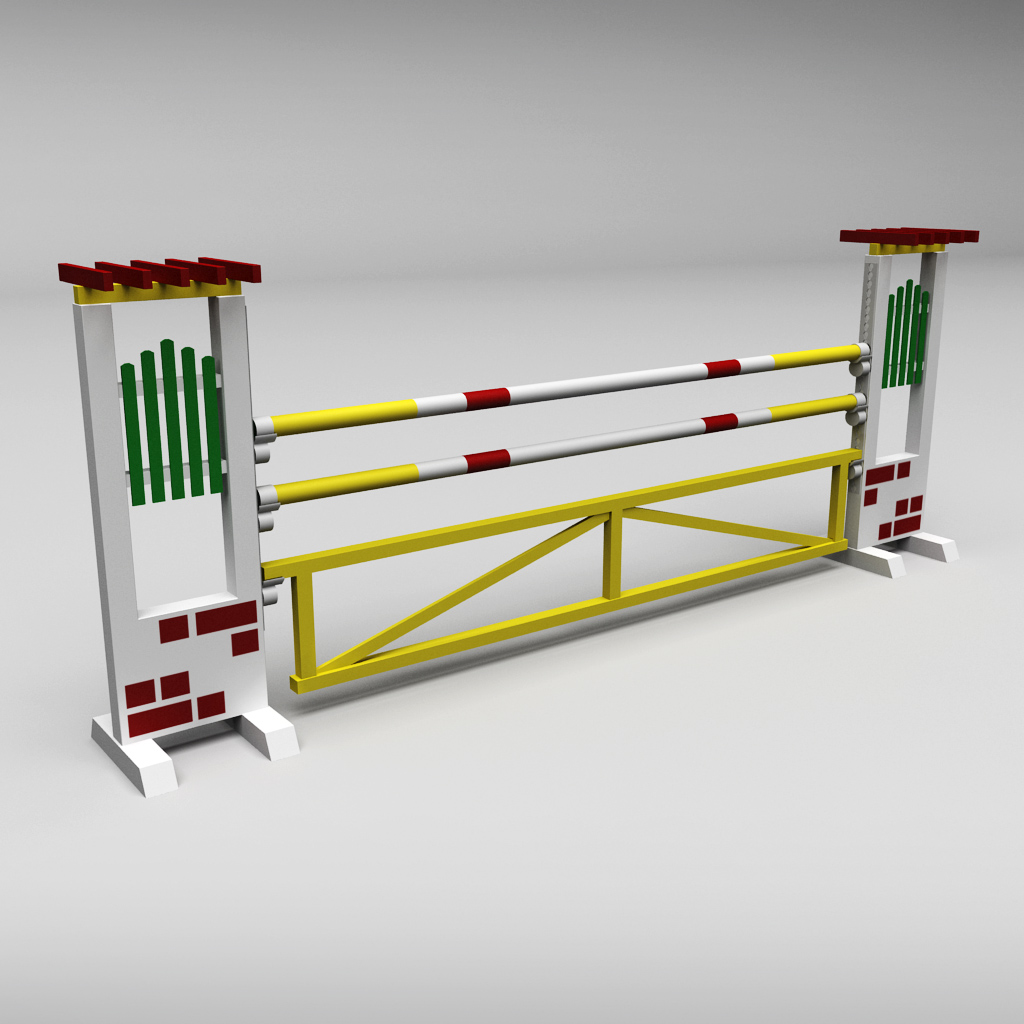This is an image of a 3D-rendered horse jump obstacle used in equestrian competitions, displayed against a plain white background. The jump setup consists of two vertical, rectangular posts on either side, primarily white with decorative elements. Each post features faux red brickwork on the lower section and a green picket-style fence within an upper window. At the top, there is a yellow decorative element adorned with red accents. The posts are connected by three horizontal components: a yellow gate at the bottom and two round bars above it, which are striped in yellow, red, and white. The gate casts a shadow on the ground, reinforcing the three-dimensional appearance of the rendering. This setup would commonly be seen in horse jumping events, either in real-life competitions or televised broadcasts.